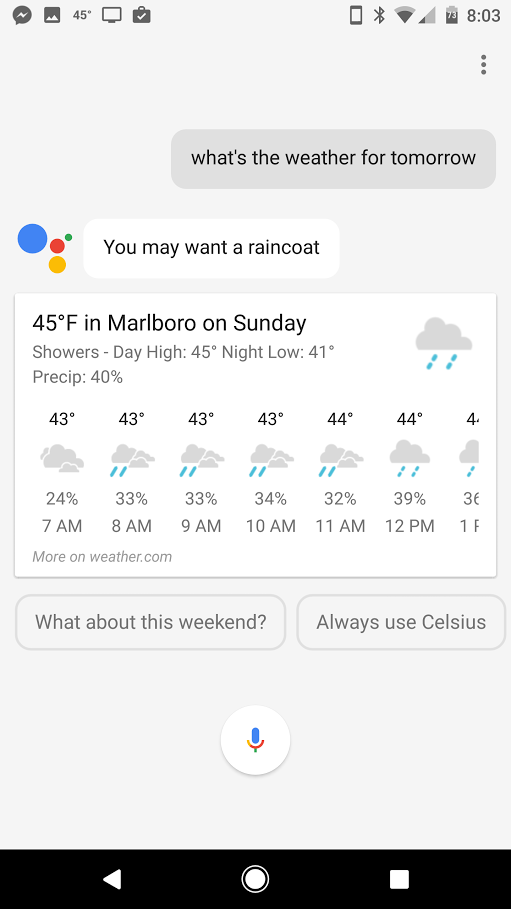This detailed and cleaned-up caption describes a screenshot of a phone screen in portrait mode. 

---

The screenshot appears to be taken from a phone. At the top left corner, there are five icons, with the third one indicating a temperature of 45°F. On the top right corner, it shows the time as 8:03 and the battery level at 73%. Directly below this on the right side, there are three vertical dots.

In the messaging app, the conversation displays a gray text reading, "What's the weather for tomorrow?" This is accompanied by an avatar that consists of a blue circle, overlayed by a red circle over a yellow circle, and a small green circle above those. A white text bubble beneath the avatar suggests, "You may want a raincoat."

Following this, a detailed weather forecast occupies a large white section. It states that the temperature will be 45°F with showers expected on Sunday. The forecast indicates a high of 45°F during the day and a low of 41°F at night, with a 40% chance of precipitation. There is an option to view more details on weather.com. Beneath the forecast are suggestion buttons for possible responses, such as "What about this weekend?" and "Always use Celsius." 

Additionally, there is a microphone icon within a white circle for voice commands. At the bottom of the screen is a prominent black stripe stretching from the left to the right. This bar includes a left-pointing triangle for going back, a white circle in the middle, and a white square at the end.

The weather forecast continues with detailed hourly temperatures for the morning, showing consistent readings around 44°F with a high probability of rain for each hour from 7 a.m. to 12 p.m.

---

This caption provides a comprehensive and detailed description of the information displayed in the screenshot.